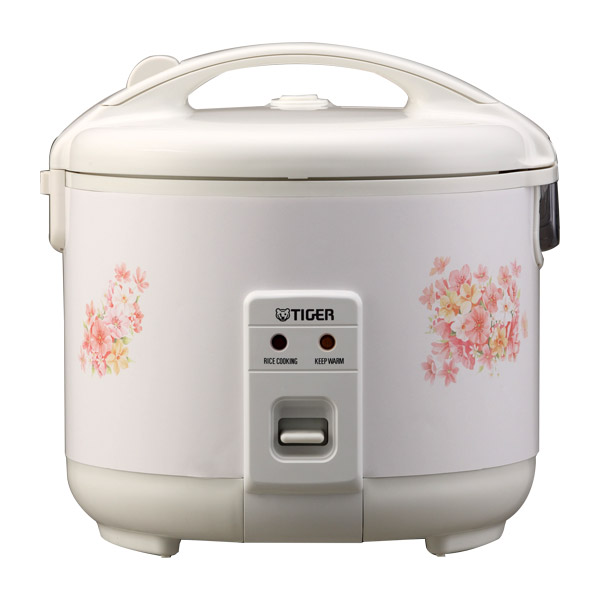This image depicts a Tiger brand rice cooker, prominently featuring the brand's logo, which includes a tiger head to the left of the control panel. The cooker is predominantly white with a round, circular design and adorned with floral patterns on both sides of the control panel. These floral designs include pink and orange flowers intermixed with smaller white flowers and green leaves, adding a decorative touch.

The control panel, centrally located on the front of the cooker, contains the text "Tiger" in black, along with two indicator lights labeled "Rice Cooking" and "Keep Warm," denoting the two available modes. Below these lights is a single knob that operates as a button to switch between the modes. 

The lid, also white, features a sturdy handle and is secured tightly with latches on either side, suggesting a pressure-sealed design for effective steaming. This lid is contrasted by a slightly off-white base and a small, possibly black component on the right-hand side, close to the handle area. The overall setting of the image against a white background gives it an advertisement-style presentation, often used for online sales or catalogs. Additionally, the rice cooker is equipped with small feet at its base for stable support.